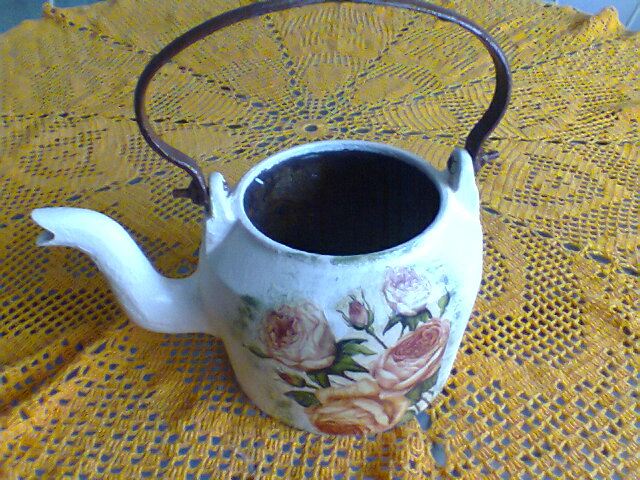The photograph captures a vintage white-painted tea kettle adorned with a hand-painted floral design featuring pink, orange, and green leaves. This charming kettle, marked by its well-worn black handle, sits upright with its spout facing left. A closer look reveals a lack of a lid, and subtle signs of aging on the handle hint at a rustic charm. It rests on a vibrant yellow paisley material, which might be a tablecloth, over a blue surface. The setting appears to be outside in natural daylight, enhancing the kettle's nostalgic allure.